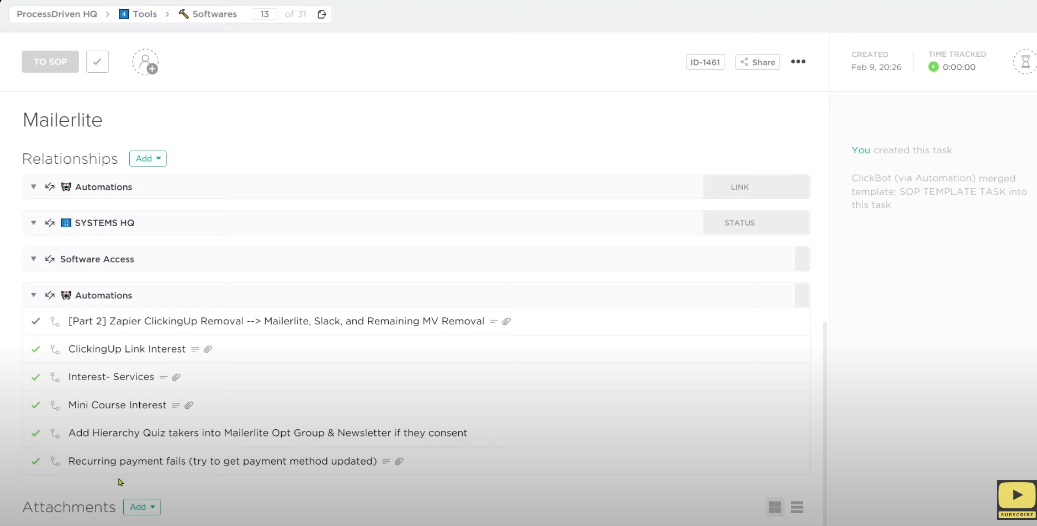In this image, a sophisticated task management interface for integrating with different systems, particularly using Mailer Lite, is displayed. The interface includes sections such as relationships, automation, system HQ, and software access. Each section is likely expandable to reveal more detailed and specific information.

On the right side of the screen, detailed information about a specific task, identified as ID 1461, is shown. This task was created by an unspecified user, with the creation date and time logged as February 9th, 2026. No time has been recorded against this task yet, as indicated by the time track set at all zeros. A green dot next to the time track suggests that the task is either ready to be activated or in the process of activation.

Additionally, there's an option at the bottom of the interface for adding attachments. This segment, labeled "Attachments," is positioned below the relationships and includes a prompt encouraging users to click to add an attachment. The attachment feature appears to be a separate, distinct area intended for additional task-related files or documents.